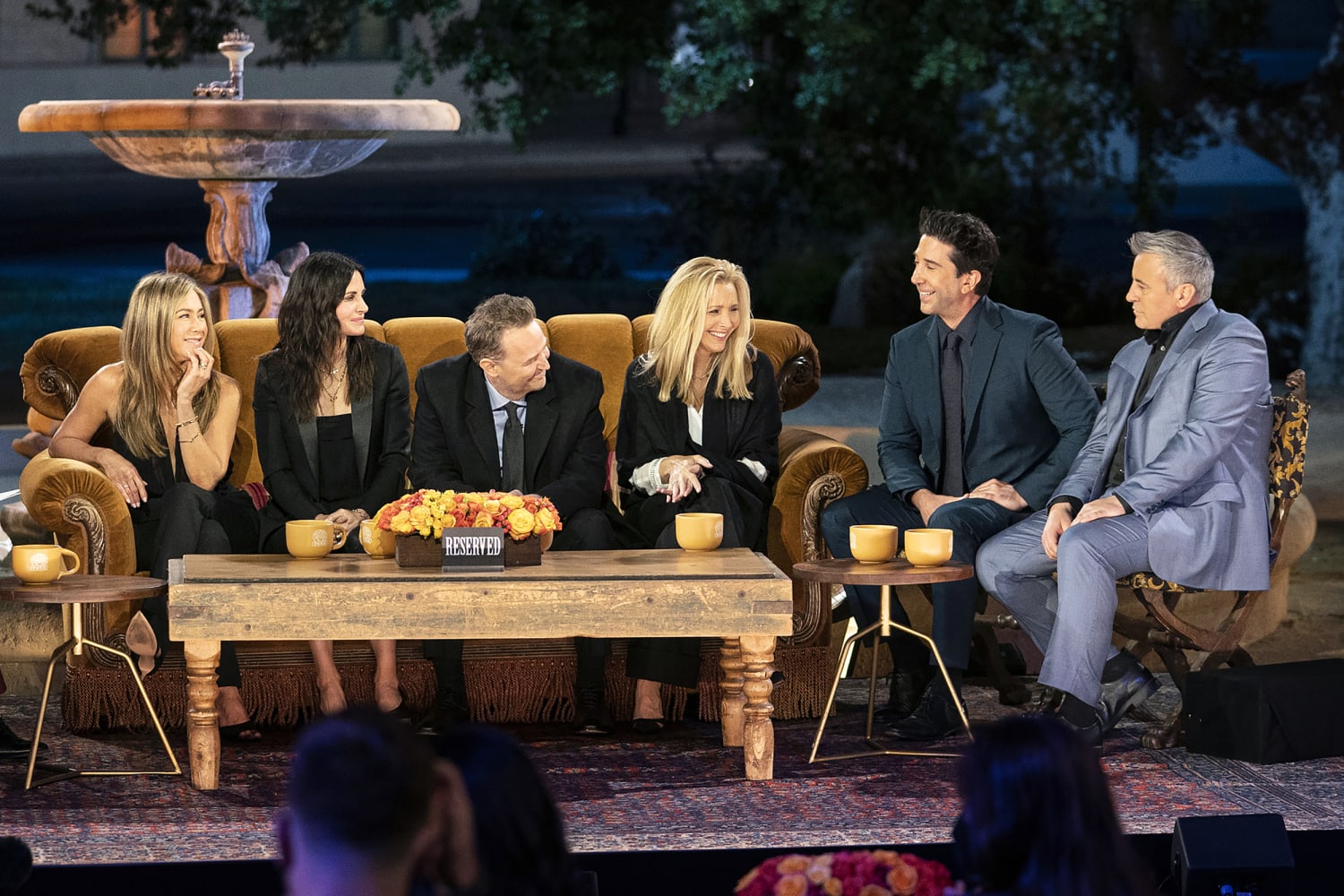This wide photograph captures a scene of a likely "Friends" reunion on stage, featuring a group of people seated around a cozy setting. In the foreground, dark silhouettes of audience members can be seen, framing the stage from below. Dominating the center of the stage is a long, velvet burnt brown couch where four adults, including Jennifer Aniston on the far left, are seated comfortably. In front of them is a small wooden coffee table adorned with a vibrant bouquet of yellow, white, and magenta flowers. 

To the right of the couch, two men occupy individual chairs positioned around a small round wooden table that prominently displays a "reserved" sign. The stage floor is covered by a striking pink and purple rug that stretches across the entire scene, adding warmth to the setup. 

In the background, the top left corner features a distinctive gray ceramic fountain that stands silently without water. To the right of the fountain, dark green trees provide a serene natural backdrop. The combination of these elements creates an inviting and intimate ambiance on stage.